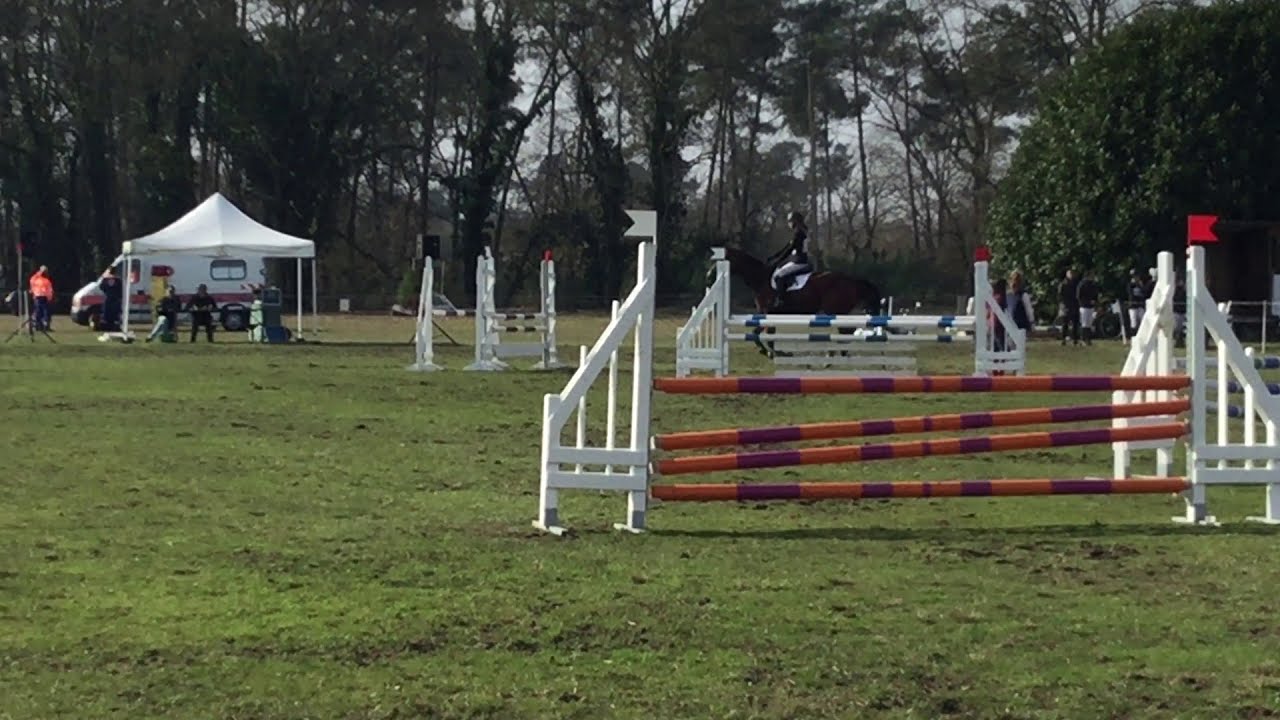The photograph captures an equestrian center set up for a jumping competition on a grassy field. In the foreground, there are white stands with red and black bars, featuring small flags on top, forming hurdles for the horses to jump over. Further back, similar hurdles with blue and white bars are visible. To the right, a black horse with a rider in full riding gear is galloping, seemingly preparing to jump. On the left side of the image, in the top corner, a white canopy tent is set up, likely for judges, with several individuals underneath, including one in a red jacket and others in dark clothing. Behind this tent is a white van with red stripes, presumably an emergency vehicle. The scene is framed by a mix of bare and leafy trees, adding a natural backdrop to this lively equestrian event.